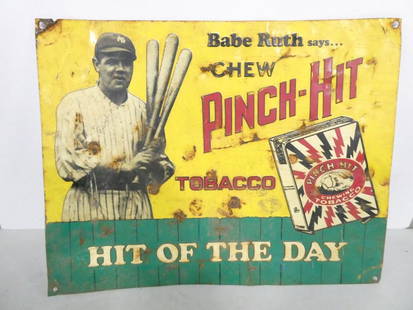This promotional advertising poster, pinned on a white wall with four silver thumbtacks at its corners, features a bright yellow upper background transitioning into a green lower section reminiscent of a picket fence. At the top, the iconic Babe Ruth, decked out in a white shirt and striped pants with a ball cap, is depicted holding three baseball bats, his image cut off around the waist. To his right, in black text, it reads "Babe Ruth says...," followed by large, bold red letters spelling out "Pinch, Hit, Tobacco." Beneath this, in white lettering against the green backdrop, is the phrase "Hit of the Day." Additionally, the poster includes a white square box with dynamic red and black lightning-bolt-like patterns converging at the center, where a red circle with a white border and a central design showcases the product, marked by the text "Pinch, Hit, Chewing, Tobacco." The upper half of the poster stands out against a yellow background, while the bottom portion complements it with green, clearly capturing the vintage aesthetic of this metal sign.